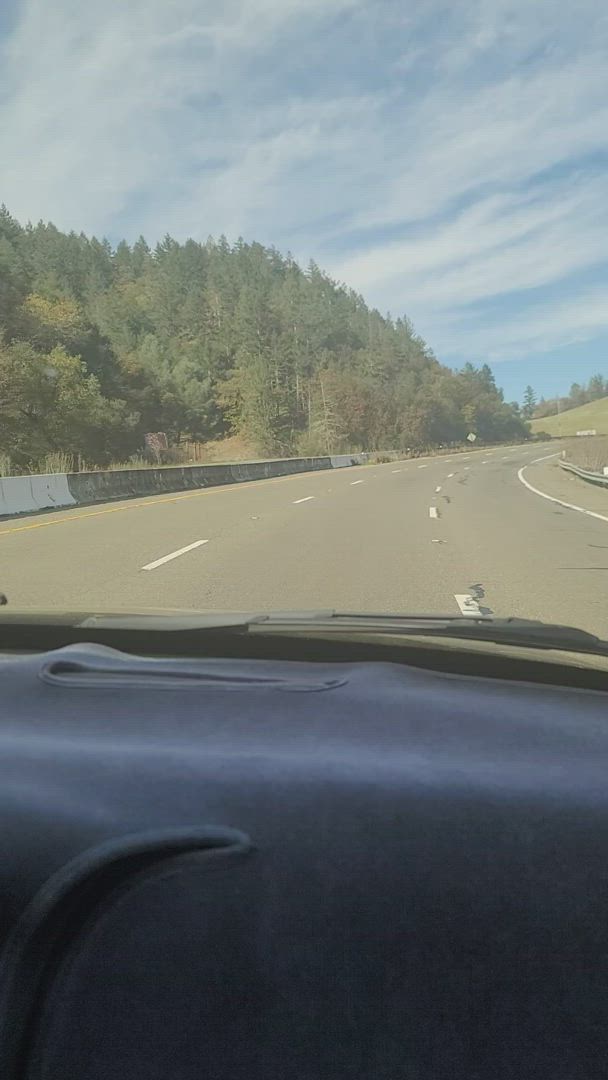This photograph, taken from the passenger seat of a car, prominently features the bottom third occupied by the car's dashboard, which is shielded with a protective fabric. The main focus is an expansive, deserted three-lane highway that gently curves to the right. On the left side of the highway, a concrete jersey barrier runs parallel, partially obscuring a dense stretch of forest that consists of various types of trees. Above, the sky is a serene blue, dotted with moderate cloud coverage. In the distant background, a hill is visible where the road subtly curves, adding depth to the scene. Notably absent are any road signs or vehicles, emphasizing the solitude and tranquility of the moment captured.